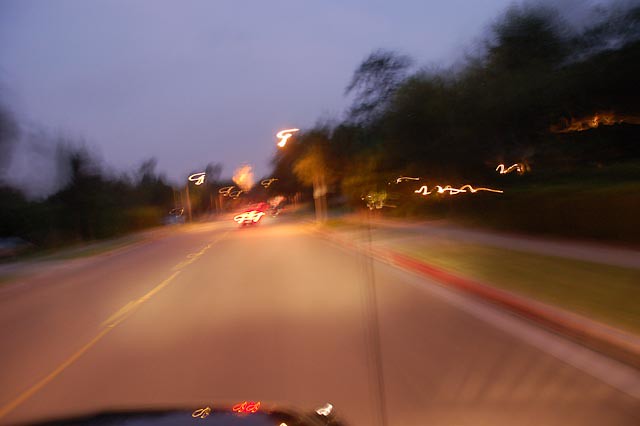Captured through the windshield of a moving vehicle, this image presents a vivid yet slightly blurred view of a road lined with trees. The vehicle travels on the right side of the road, which is marked by a solid white or yellow median line running down its center. Street lamps, either hanging or mounted on tall poles, illuminate the scene, casting vibrant, squiggly lines of light against the blur from the glass. This effect creates a dynamic, almost abstract composition. Both sides of the road feature grass boulevards and sidewalks, with the right side showing hints of a hedge that might belong to a nearby residence. The combination of motion blur and fluorescent lighting gives the image an energetic and surreal quality.